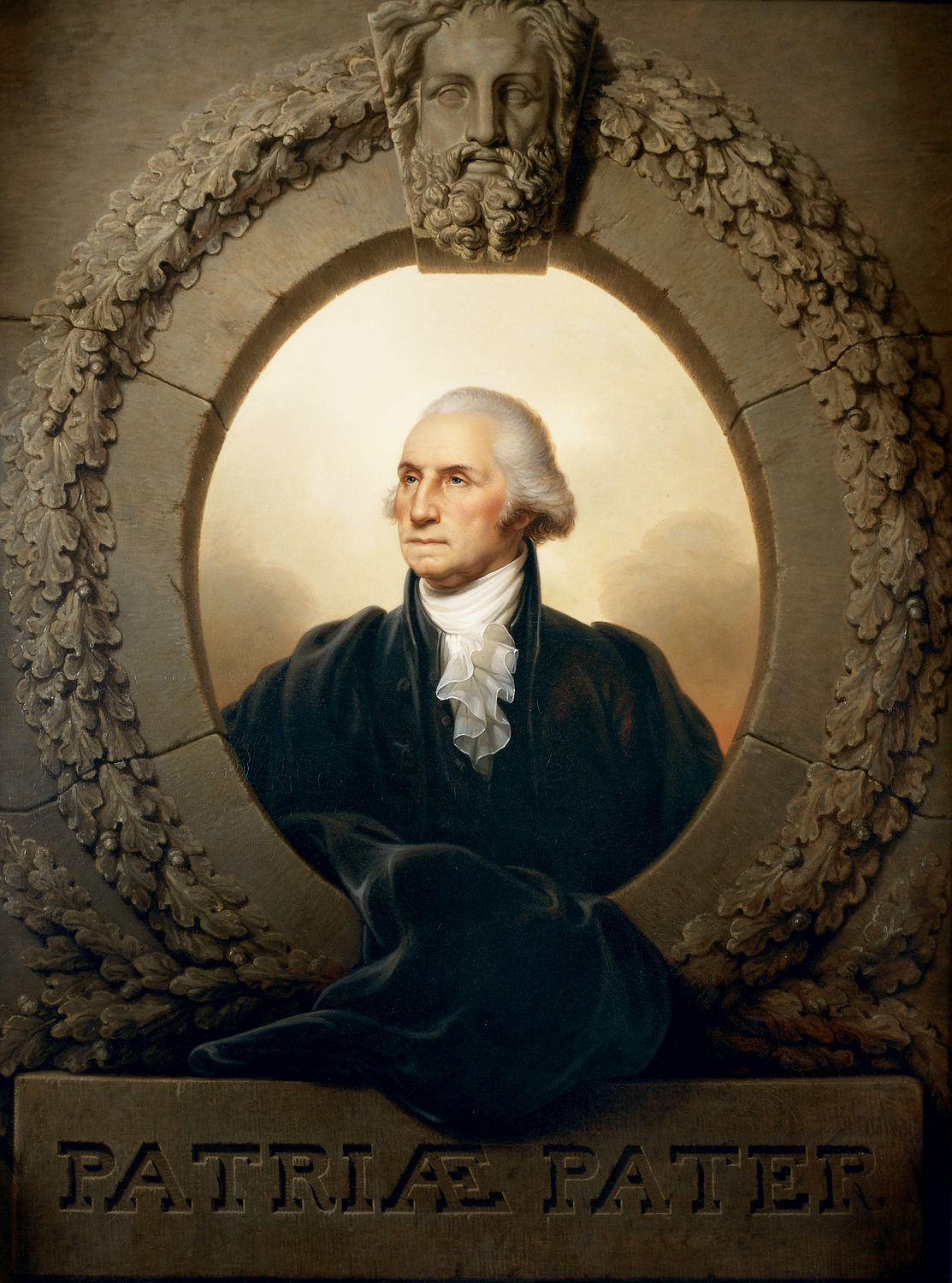The image is a detailed and intricate portrait of General George Washington, set within a majestically carved frame mimicking ancient Roman or Greek art. At the top of the frame is a depiction of a Greek god, possibly Zeus, rendered in a tan stone. Surrounding the oval frame are meticulously crafted laurel leaves, reinforcing the classical theme. Washington, wearing his recognizable black coat over a traditional white ruffled shirt, commands the center of the portrait, his hair styled back and his gaze seemingly directed upwards. Intriguingly, the lower part of his coat flows out of the oval frame, creating a 3D effect as it rests on a rectangular base below. This base is inscribed with the Latin phrase "Patriae Pater," which translates to "Father of the Fatherland."